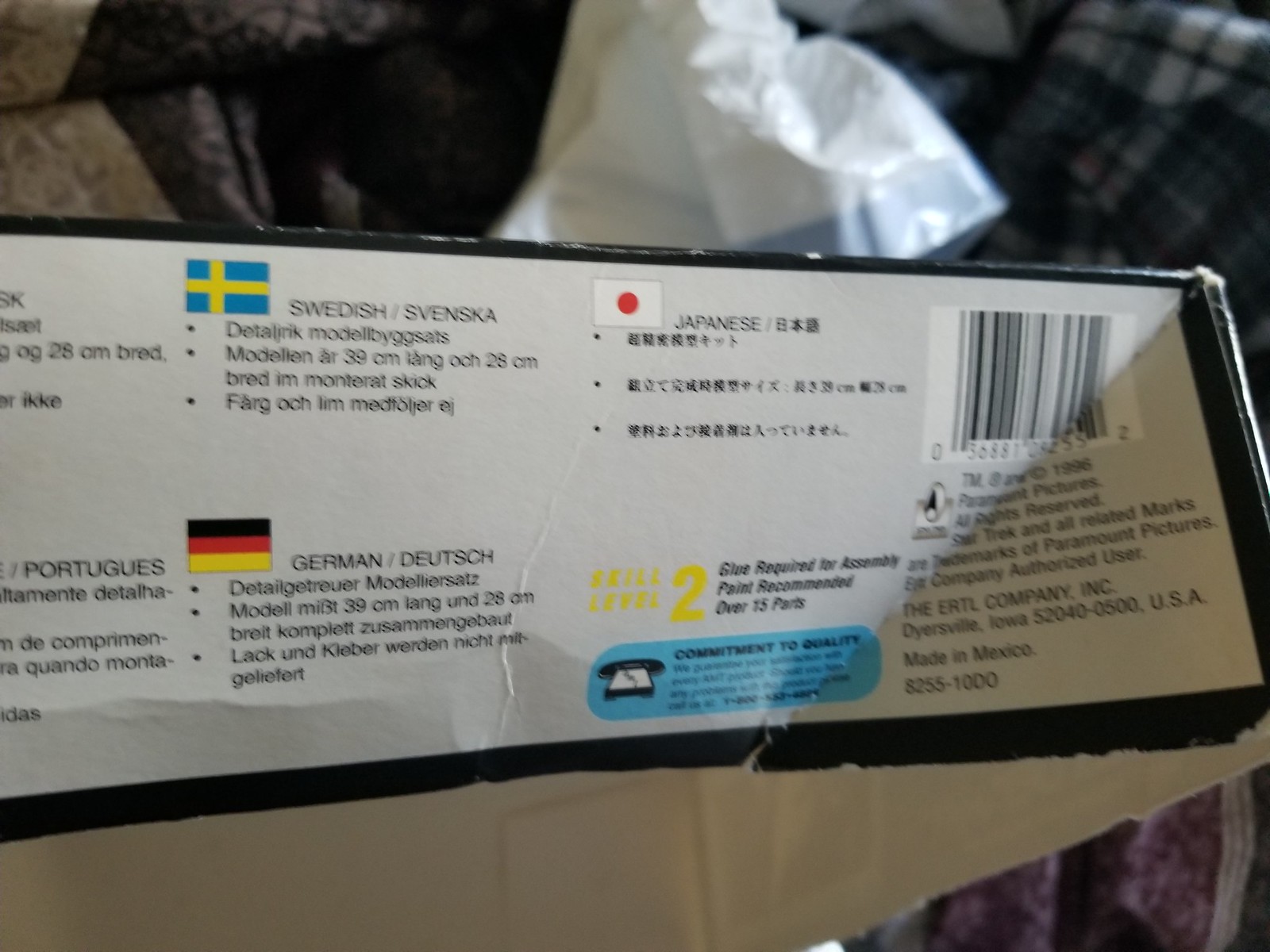In the image, we observe a partially opened box displaying a variety of informative details. The visible side of the box features the flags of Sweden, Japan, and Germany. Prominently marked with a yellow "2," the box also presents a barcode to the right. The manufacturer's name, "Ertl," is clearly printed, along with a note indicating the item was made in Mexico. Additional information on the box suggests that it may be a model kit, as it specifies that glue is required for assembly, paint is recommended, and the kit contains over 15 parts. The image leaves the contents inside the box unknown, adding an element of intrigue.